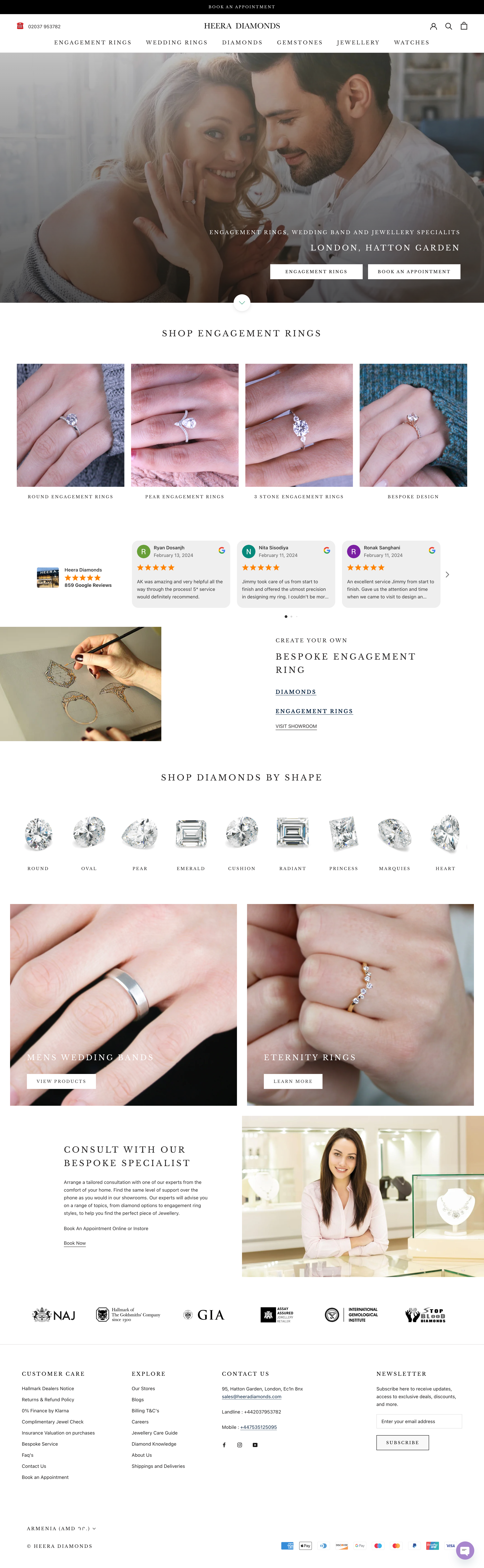This image captures a detailed web page advertisement for Heera Diamonds, prominently featuring engagement rings and luxury jewelry. At the top, there's a header with options for Engagement Rings, Wedding Rings, Diamonds, Gemstones, Jewelry, and Watches, alongside a cart and search feature. Beneath the header is a large photograph of a smiling couple: the woman on the left, showcasing her engagement ring with her blonde hair and fair-tan skin, dressed in an off-the-shoulder gray shirt, while the man stands to her right, wearing a white shirt and looking down at the ring. This section is labeled "Engagement Rings, Wedding Band, and Jewelry Specialist, London Hatton Garden," with a phone number and a 'Book an Appointment' button.

Below this couple’s image are four high-resolution, close-up photographs of different engagement rings on women's hands, emphasizing various diamond shapes and styles. Following these images, an artist is depicted meticulously sketching an engagement ring, including the diamond and band details. This illustration underscores the customization and craftsmanship of the rings.

Further down, there are gray logos and labels detailing the types and shapes of diamonds available, including round, oval, pear, emerald, cushion, radiant, princess, marquee, and heart. This segment is succeeded by another set of two photographs showcasing more women's hands adorned with diamond rings.

The webpage continues with a photograph of a woman standing at a table, arms crossed, beside a diamond necklace display. The bottom of the page includes various resources and text sections labeled Customer Care, Explore, Contact Us, and Newsletter, providing comprehensive customer information and support options. The prevalent colors in the imagery are flesh tones, whites, browns, and grays, contributing to an elegant and sophisticated aesthetic.